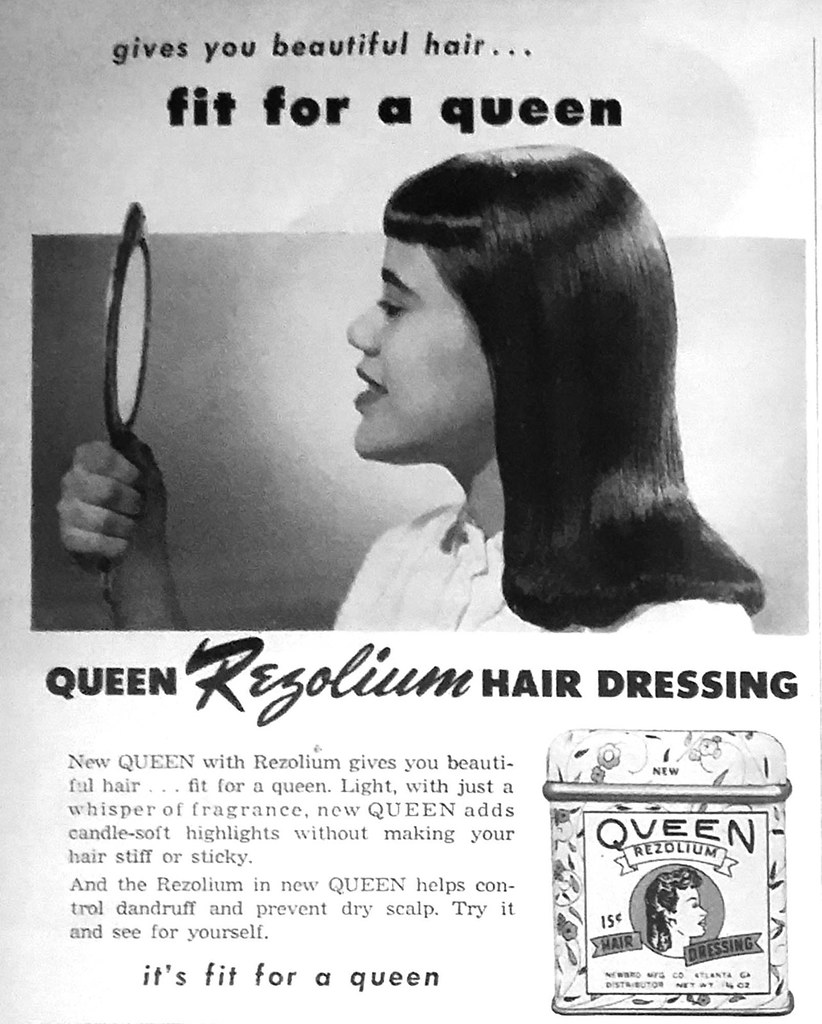This is a vintage black-and-white advertisement, likely from a magazine, promoting Queen Rhizolium Hairdressing. At the center of the ad, an African American woman with shiny, smooth black hair cascading to her shoulders is depicted. She is wearing a white high-neck blouse and holding a handheld mirror with a black rim in her left hand, looking into it with a smile. Above her, the text reads: "Gives you beautiful hair... fit for a queen."

Beneath the main image, there's a detailed paragraph extolling the product's virtues: "New Queen with Rhizolium gives you beautiful hair, fit for a queen. Light with just a whisper of fragrance, New Queen adds candle-soft highlights without making your hair stiff or sticky. And the Rhizolium in New Queen helps control dandruff and prevent dry scalp. Try it and see for yourself."

Further down, in larger text, it emphasizes: "It's fit for a queen." On the right side of the ad, there's an illustration of the product—a rectangular tin canister adorned with a flower pattern and a white label that reads "Queen Rhizolium." Beneath this, another illustration of a woman with long black hair facing right is shown, along with the product's affordable price: "15 cents Hairdressing."